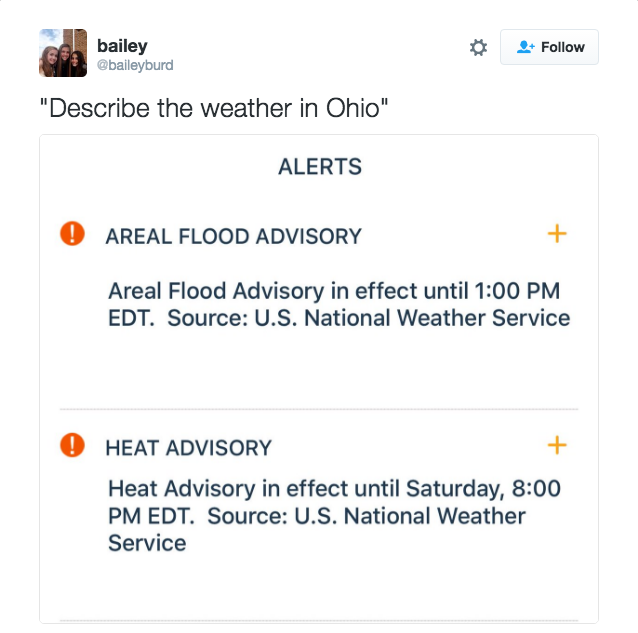The image is a screen capture of a Twitter web page, prominently featuring a user profile. In the top-left corner, there is a profile picture of three girls. To the right of the profile picture, it shows the username "Bailey" and the handle "@BaileyBird". Adjacent to this are two buttons: a settings icon and a follow button.

The rest of the page has a white background with black text, organized into three distinct sections. The first section is a single line that reads, "Describe the weather in Ohio," enclosed in quotes.

Beneath this line are two gray-bordered boxes containing weather alerts. The first box, marked with a circle containing an exclamation mark, carries an "Aerial Flood Advisory". The detailed text within this box states: "Aerial flood advisory in effect until 1 p.m. EDT. Source: U.S. National Weather Service." There is a plus sign in the upper right corner of this box, indicating an option to expand for more details.

The second box, marked with a red circle containing an exclamation mark, includes a "Heat Advisory". The text specifies: "Heat advisory in effect until 8 p.m. EDT on Saturday. Source: U.S. National Weather Service." Similar to the first box, a plus sign in the upper right corner allows expanding for further information.